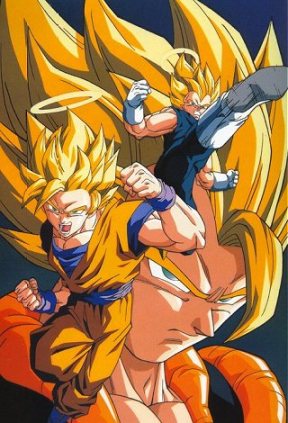A detailed depiction of an anime-inspired illustration showcases a dynamic character from multiple perspectives. Dominating the composition is a large profile view of a Caucasian individual, distinguished by his spiky blonde hair, which serves as the central focus of the artwork. Flanking this primary image are two smaller, action-packed vignettes of the same character. 

In the top section, the character executes a powerful high kick with his right leg, exuding agility and martial prowess. Below, donned in a striking yellow gi, he delivers a formidable punch, suggesting his involvement in martial arts. Both action scenes are accentuated with ethereal halos, adding a sense of emphasis and energy to the character’s movements. The combination of these elements forms a cohesive and visually engaging portrait, capturing the essence and dynamism of a martial artist in an anime or manga style.